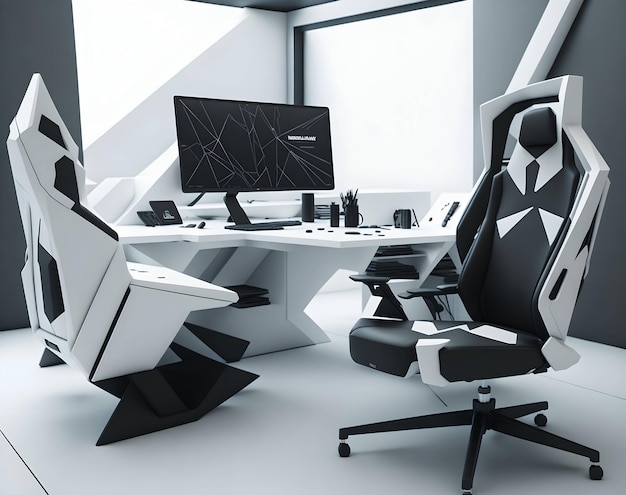This black and white image portrays a highly modern and futuristic workspace, resembling a sophisticated gaming setup. The room features sleek, angular designs throughout, with white walls accentuated by sharp black and white geometric patterns. Central to the space is a T-shaped, all-white desk with storage compartments underneath, hosting a large black computer monitor. The desk is also adorned with black and gray accessories, including a pencil holder, a frame, and an assortment of small, indistinct items.

Two distinctive chairs are positioned at the desk, both exhibiting a contemporary, almost space shuttle-like appearance. One chair boasts a dual-tone black and white design, characterized by a thick, modern edge outlining its back, and is equipped with wheels for mobility. The other chair features a hard plastic exterior that culminates in a pointed top, with a base structured from straight lines, giving it a non-traditional, possibly rocking, capability. The room's floor is white, enhancing the minimalist yet highly stylized ambiance of this futuristic office setting.